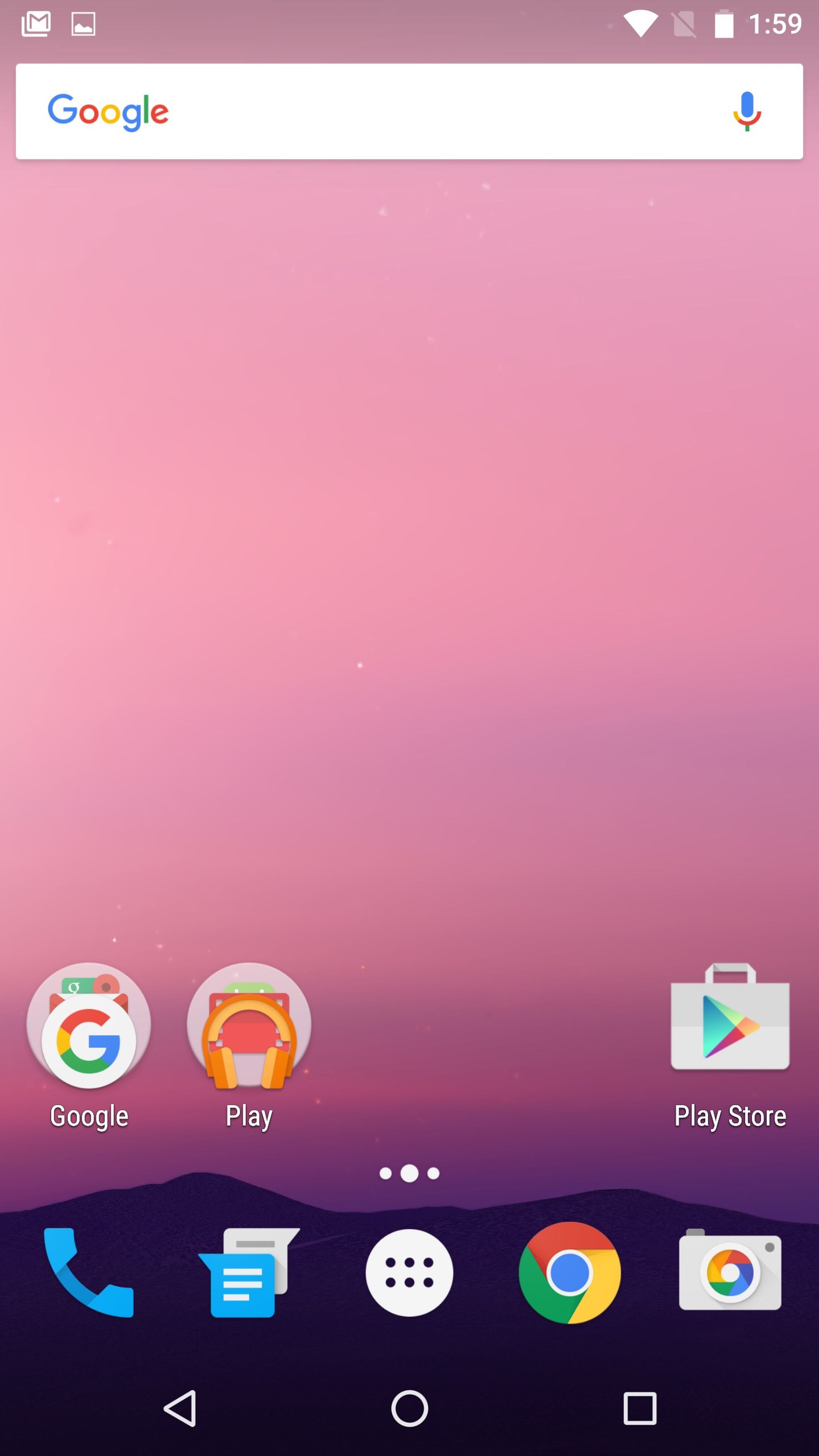This image is a detailed screenshot of a smartphone's home screen. At the top of the screen, from left to right, a set of status icons include a picture symbol, a Wi-Fi indicator, a symbol that appears to be X'd out with a bar through it, a battery icon, and the current time displayed as 1:59. Below these icons sits a search bar featuring the Google logo, with each letter colored differently (blue, red, yellow, and green). On the right side of the search bar, there is a microphone icon, which allows for voice input.

The background of the screen exhibits a gradient, starting with a vibrant pink at the top which gradually transitions into a deep purple towards the bottom. Overlaying this gradient are silhouettes of dark-colored mountains, adding a scenic touch to the backdrop.

Prominently displayed on the home screen are several icons. From left to right, these include the Google icon, a Google Play icon represented by headphones, the Google Play Store icon depicted as a shopping bag featuring the Google logo, and there are other essential app icons such as a phone, a messaging app, a circular icon with six dots representing the app drawer, the Google Chrome browser icon, and another Google icon identified as the camera app.

At the very bottom of the screen are the navigation buttons: a left-facing arrow for back, a circle for home, and a square for recent apps. These buttons provide easy access to essential functions of the device.